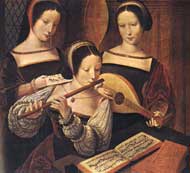This is a detailed color illustration, possibly from the medieval or Renaissance period, depicting three pale-skinned women with dark hair, all dressed in old medieval or early-period attire. The central figure, seated at a round table, is engrossed in playing a flute while looking down at sheet music spread out in an open book. Behind her left shoulder stands a young woman with long, flowing black hair, who appears to be examining an unclear white object in her hand. To the right, another young woman with dark hair pulled back and adorned with a headband is seen playing a lute. The scene, painted with intricate detail, captures a moment of musical collaboration among the three women.